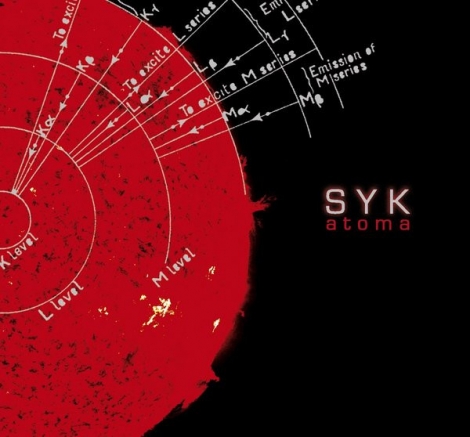The image is a detailed and stylized graphical design, likely representing a scientific diagram or possibly the cover of a music album. It features a large, circular red object dominating the left side of the image, resembling a sun or a red star, with filaments and solar flare-like spikes emerging from its edge. This circular object also contains black blotches and is overlaid with concentric light gray or white circles. These circles are annotated with various labels such as "K level," "L level," and "M level," with additional white lines extending from them, culminating in arrows and more text, suggesting regions or layers within the star. The background is completely black, enhancing the vivid maroon, red, gray, and white colors of the primary object. On the right side of the image, there is white text reading "SYK" in capital letters on one line and "ATOMA" in red lowercase letters on the line below. This text appears isolated against the black background, balancing the composition and contributing to the overall diagrammatic style of the image.